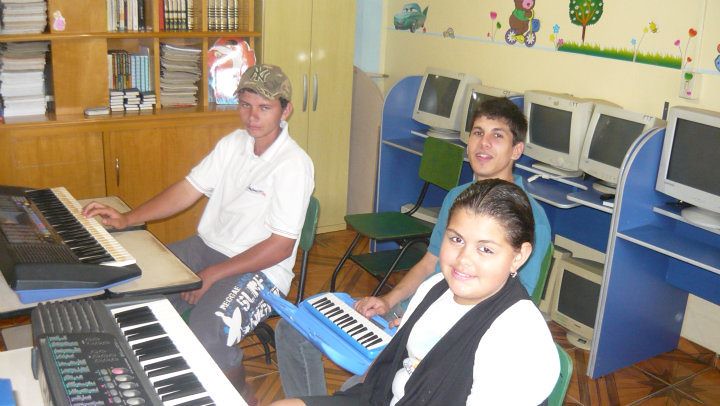The photograph depicts a classroom setting, likely taken 10 to 15 years ago, with a wooden floor and beige walls adorned with colorful children's drawings, including one of a girl riding a bike surrounded by flowers. In the forefront are three students, vertically aligned and facing the camera. The student in the middle, wearing a blue shirt, holds a blue and white keyboard on his lap. To his left, a girl in a white shirt with a gray vest also has a larger black and white keyboard in front of her, and to his right, another student in a white t-shirt and gray sweatpants is playing a keyboard placed on a tray. The background features a brown bookcase filled with books and several old computer monitors, emphasizing the room's multifunctional use, potentially as a computer or music room. The blue stalls at the back add to the classroom ambiance.